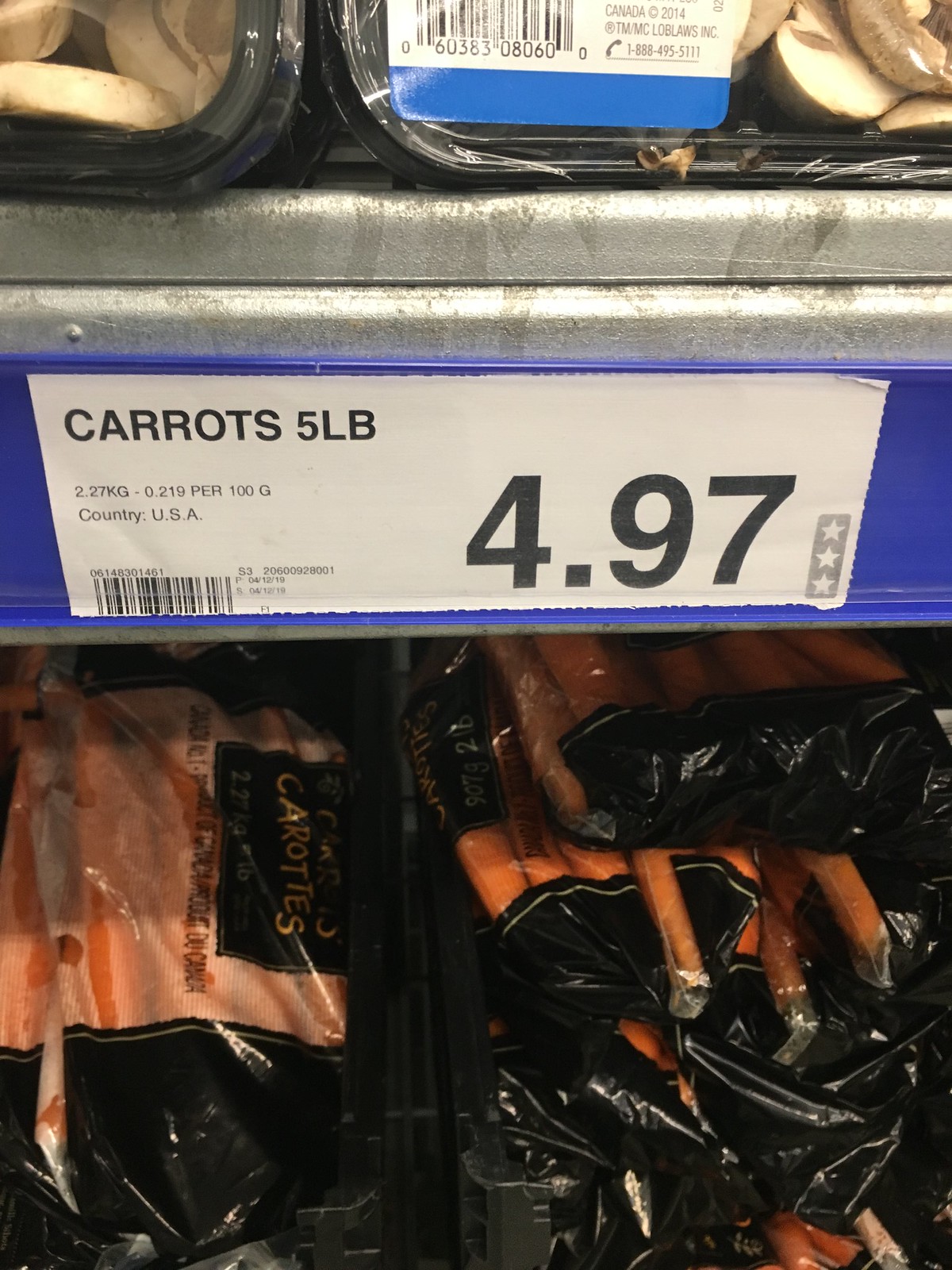On a sturdy, thick steel shelf, a variety of vegetables are displayed. The top shelf is laden with fresh mushrooms, while the bottom shelf showcases large bags of carrots. The carrots are prominently labeled with a sign featuring a blue background and white text. The sign reads "Carrots, Five Pounds," priced at $4.97. Each bag of carrots is substantial, with a black label indicating the contents and weight. The large quantity suggests that this display is in a warehouse store, likely Costco.